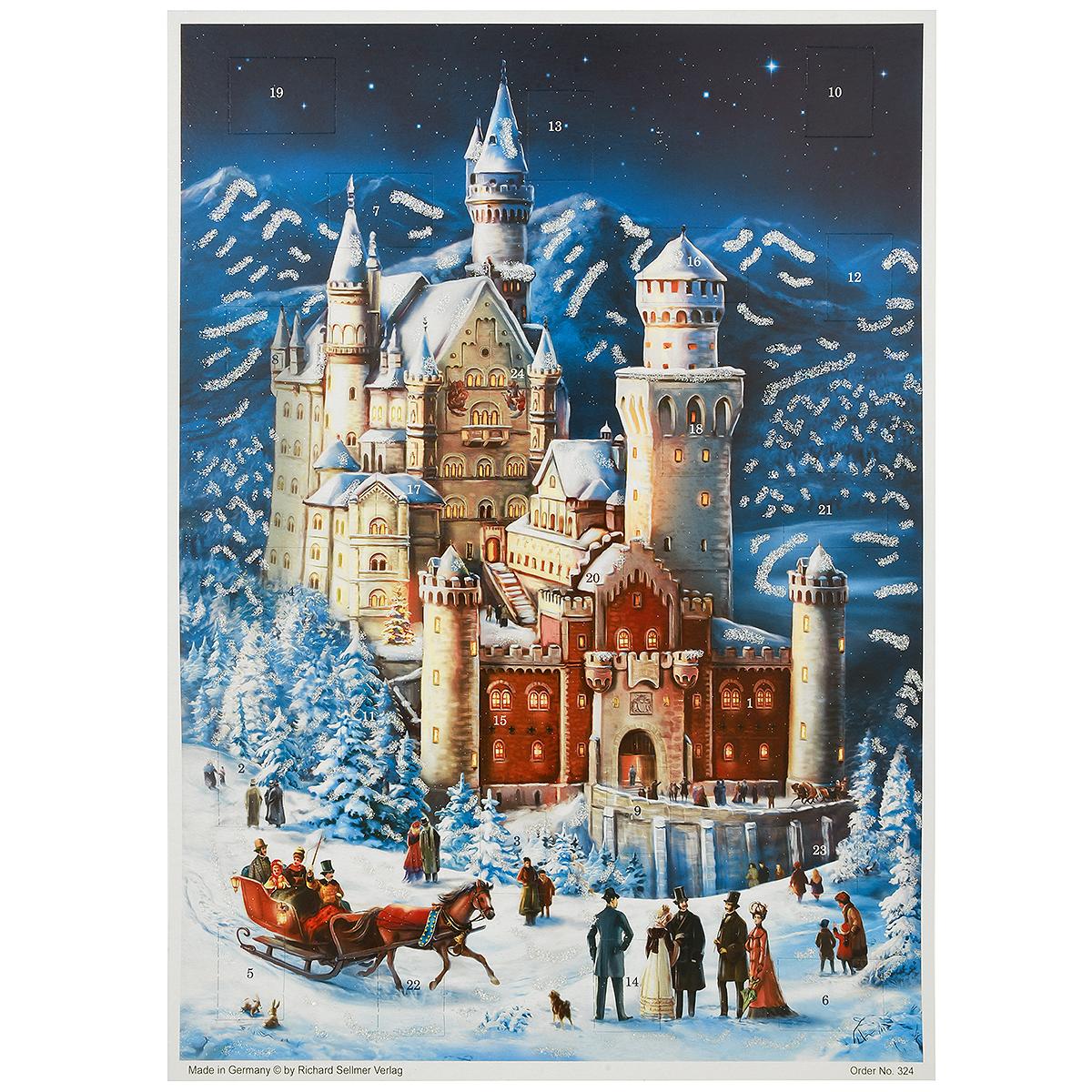The image depicts a beautifully illustrated winter scene reminiscent of a classic Christmas card. At the heart of the image stands a grand, red castle adorned with numerous cone-shaped towers, surrounded by a series of snow-capped trees and smaller white buildings. Mountains, dusted with snow, rise majestically in the background against a black and blue sky, providing a striking contrast to the warmth of the reddish-brown and green hues in the foreground. The snowy foreground is lively with an assortment of people engaging in winter activities; to the lower left, figures gather near a dog while further inwards, a horse pulls a sleigh filled with people. The entire scene is bordered by a subtle gray frame. Notably, this picturesque artwork is a holiday card made in Germany, copyrighted by Richard Selman Verlag, order number 324. It combines elements of traditional winter charm with bustling human presence, encapsulating the festive spirit of the season.